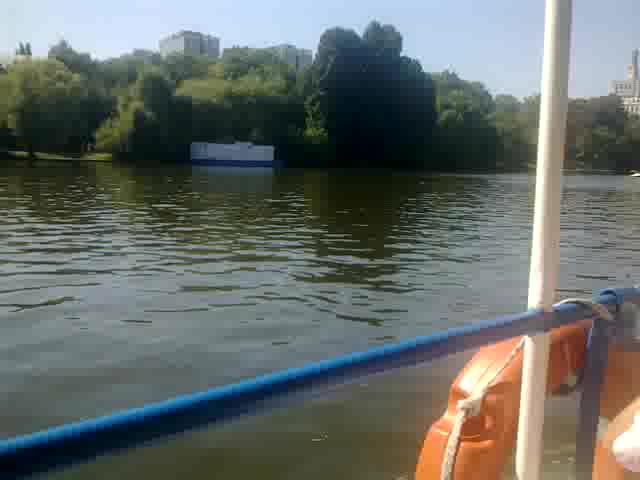The image depicts a tranquil scene taken from a boat on a wide river. Dominating the foreground is a blue railing, accompanied by a vertical white bar and an orange life preserver. The river appears calm, its murky green hue reflecting the day's light under a soft blue sky. In the background, lush, fully-leafed green trees frame the scene, obscuring distant branches. Among the foliage, a large, dark green tree stands out, likely due to the way sunlight dapples its neighbors. Nestled at the water's edge, a small white rectangular structure with a blue base suggests a houseboat. Further in the background, partially concealed by the trees, is a square, castle-like building, enhancing the picturesque quality of the landscape. The water exhibits gentle ripples, completing this serene riverside vista.